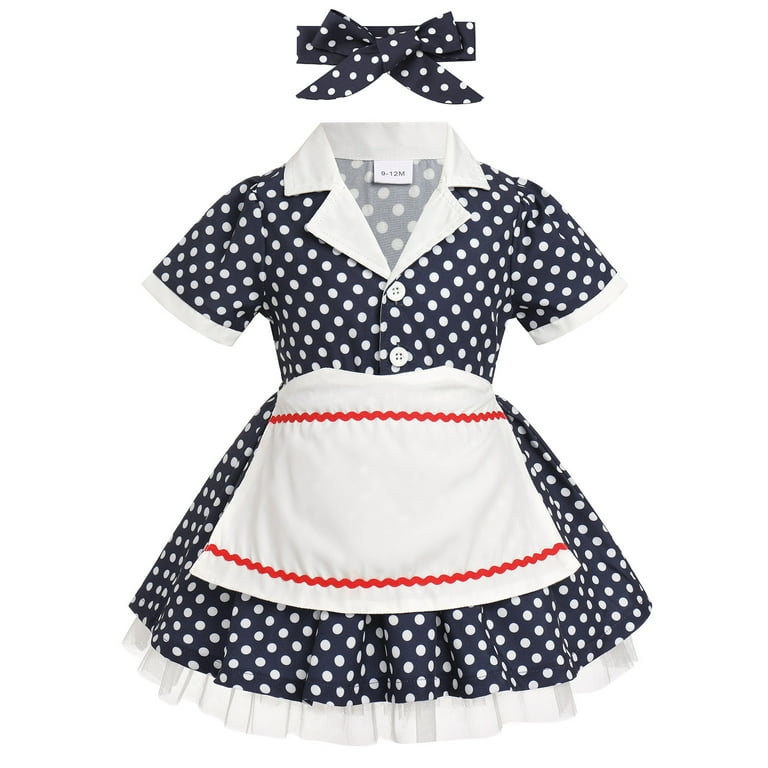This is an image of a retro 1950s-style waitress costume, reminiscent of the mid-20th century. The ensemble features a short-sleeved dress with a dark navy blue or black background adorned with white polka dots. The dress is detailed with a defined white collar, white piping around the sleeves, and large white buttons down the front. It cinches at the waist and ends with a charming white ruffle or petticoat at the hem.

Adding to the nostalgic charm, the outfit includes a simple white apron. The apron, tied around the waist, is decorated with red rickrack along the top edge and the bottom hem, providing a striking contrast to the dress. Completing the look, there's a matching headband—a ribbon with a bow—that mirrors the dress's polka dot pattern. This delightful costume evokes a sense of vintage elegance and could easily be imagined in a 1950s-style restaurant setting.